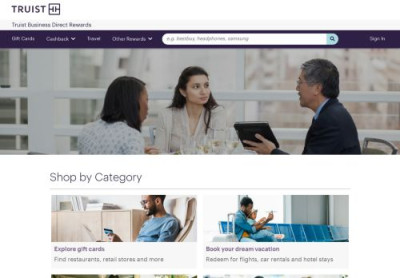A screenshot of the Truist website's top section features a distinctive layout. At the header's top, "Truist" is prominently displayed in purple, accompanied by a square purple logo on its right. This is followed by a light gray navigation bar containing text aligned to the left. Beneath this, there's an illegible purple bar that includes four menu options, along with a pill-shaped search bar and a sign-in button on the far right.

Directly under this purple bar, the main banner image captures a scene with three individuals seated at a table. On the left, a Black woman and a tan-skinned woman are engaged in conversation with a tan-skinned man who has gray, salt-and-pepper hair, seated to the right. The man is holding a tablet in his left hand, implying a discussion of technological or financial matters.

Below this banner image, the website's content is organized into categories, each represented by two different images with text descriptions underneath. This section features a clean, white background that enhances readability and visual appeal.